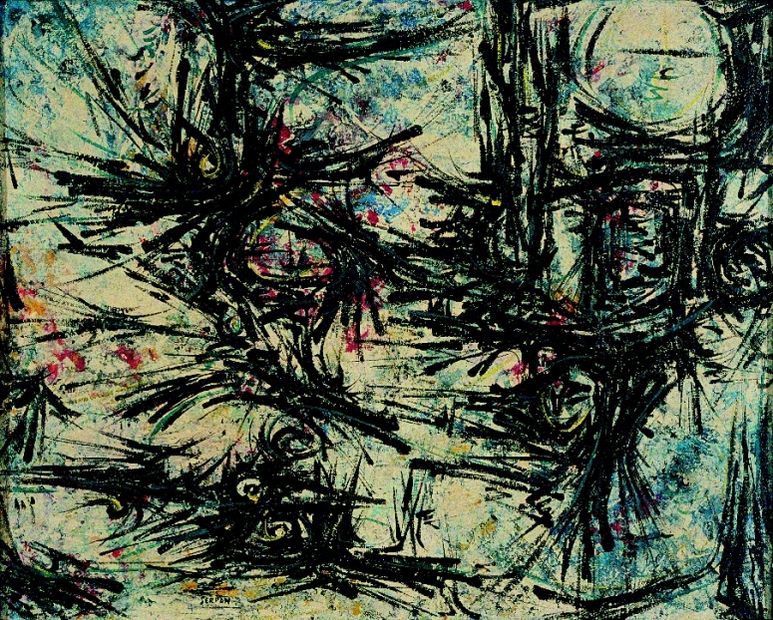The image is an abstract painting featuring a chaotic array of thick black paint strokes and lines against a gradient background that transitions from light to dark green, interspersed with hues of yellow, blue, and red. These black lines are prominent and dominate the composition, appearing in clusters and forming various shapes. Some bundles of lines resemble sticks grouped together, while others take on circular or curved forms, creating an intricate pattern across the canvas. The background, initially a white canvas, is now faintly visible through the splotches of color and layered black paint, adding texture and depth to the artwork. Overall, the piece showcases two dominant columns of abstract shapes, with the left side featuring three distinct forms, and the right side presenting an upside-down house-like shape, making the entire composition a dynamic and visually intense abstract painting.